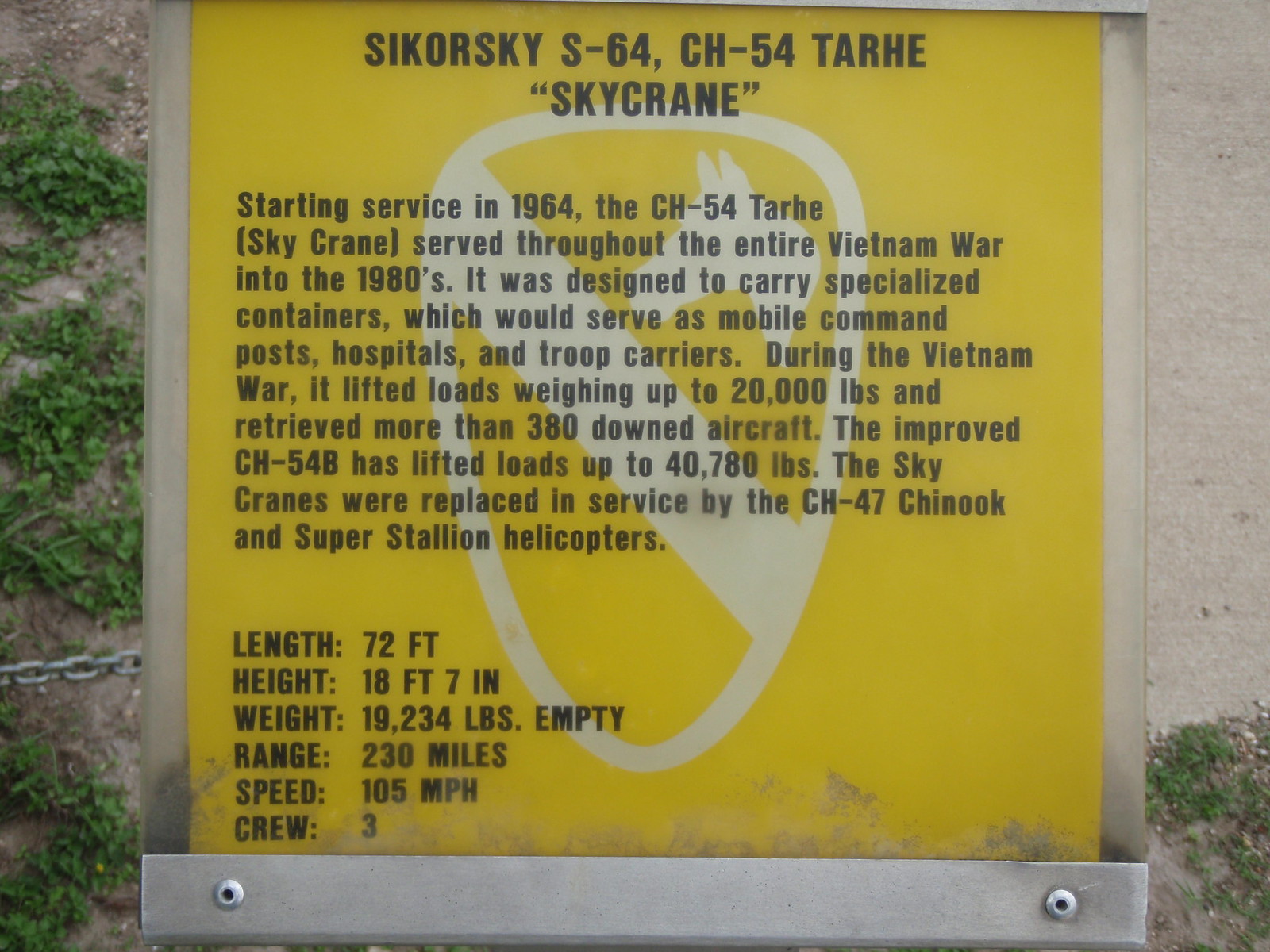The image features a yellow metal placard with a central shield design, showcasing black text that reads "Sikorsky S-64 CH-54 'Tar Hei' Sky Crane." This helicopter began its service in 1964 and played a crucial role throughout the Vietnam War until the 1980s. Designed to carry specialized containers, it functioned as mobile command posts, hospitals, and troop carriers. During the Vietnam War, the Sky Crane demonstrated its capability by lifting loads weighing up to 20,000 pounds and retrieving more than 380 downed aircraft. The enhanced version, CH-54B, could lift loads up to 40,780 pounds. Ultimately, the Sky Cranes were replaced by CH-47 Chinook and Super Stallion helicopters. The placard also provides detailed specifications: a length of 72 feet, a height of 18 feet 7 inches, an empty weight of 19,234 pounds, a range of 230 miles, a speed of 105 miles per hour, and a crew of three.